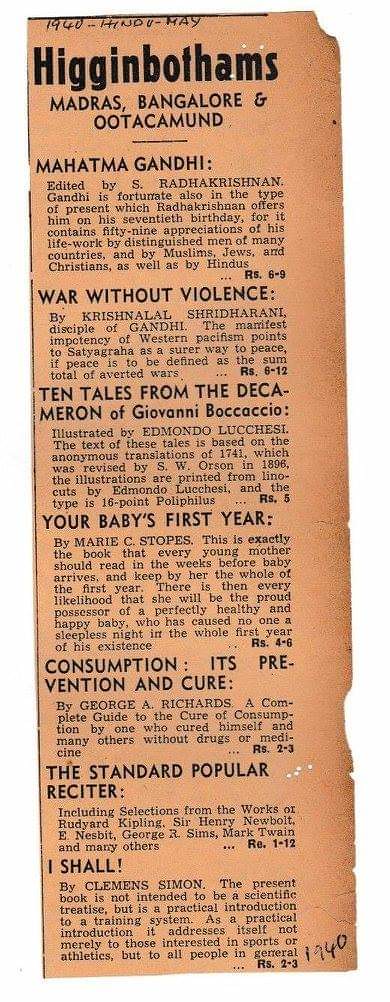This image shows a section of an old, reddish-pink colored newspaper dated May 1940. At the very top of the page, it reads "1940 Hindu May." Below this heading, the large, bold title "Higginbothams" is prominently displayed in black, followed by the locations "Madras, Bangalore, and Uttakamund." The column is divided into several sections, each with their own title and accompanying text that is too small to read clearly. The sections are titled: "Mahatma Gandhi," "War Without Violence," "Ten Tales from the Decameron of Giovanni Boccaccio," "Your Baby's First Year," "Consumption, Its Prevention and Cure," "The Standard Popular Reciter," and "I Shall." The text under each of these titles is also too small to decipher.